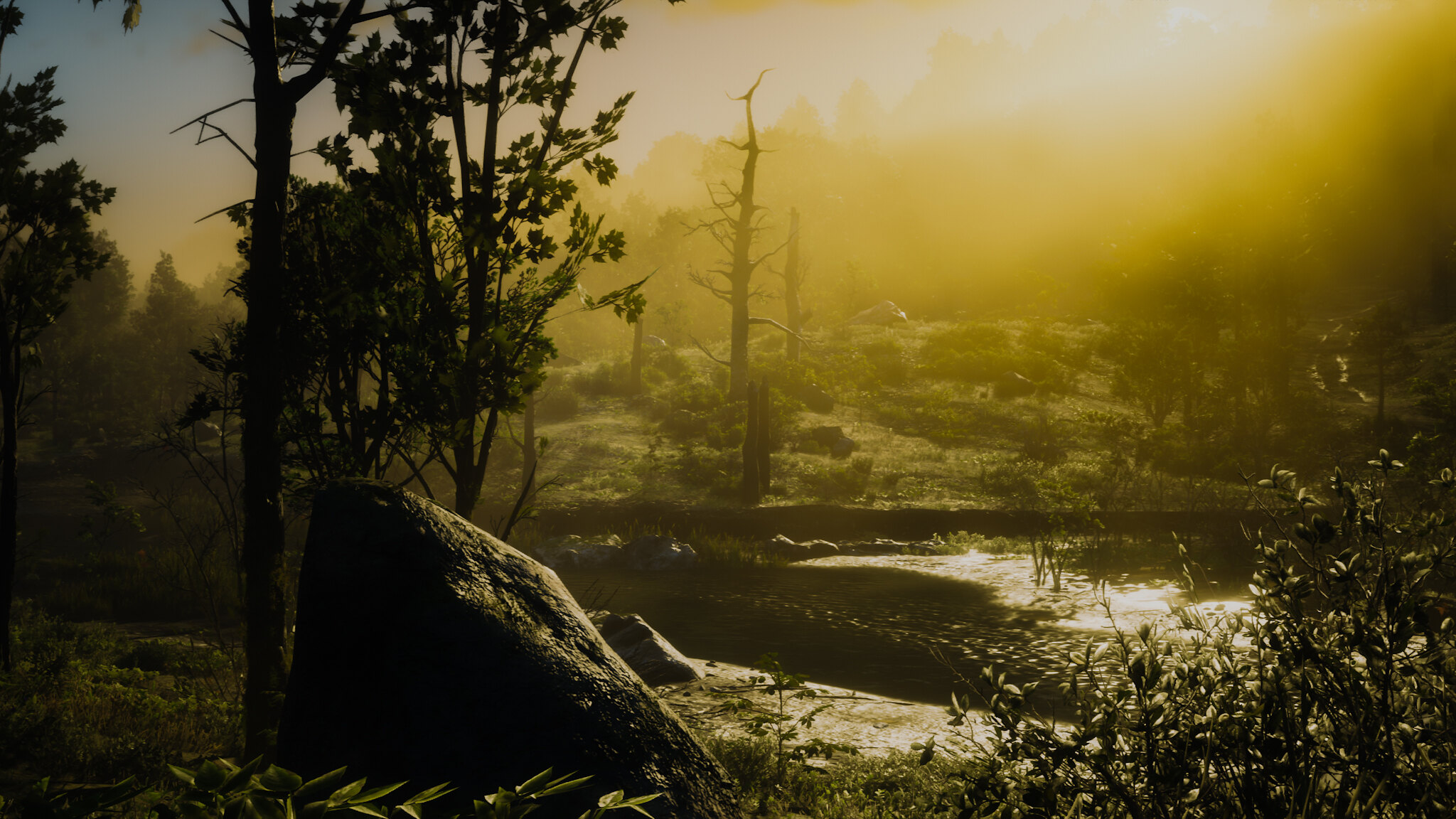This image is a highly detailed, possibly AI-generated, artistic rendering of an outdoor scene showcasing a serene, possibly forested landscape during sunrise or sunset. The sun is positioned in the upper right-hand corner, casting a brilliant yellow light across the scene, illuminating the tops and right sides of the trees, and creating distinct highlights on a large, triangular rock located in the lower center-left part of the image. The rock, beautifully drawn with intricate shadows, sits near the most prominent tree and is flanked by a bush or shrub with succulent-like, pointy leaves on the right side. The scene features a gently rolling grassy or dirty area extending from the far side of a stream or small river that ambles through the lower third of the image, identifiable by the reflective highlights on the water's surface. The background is shrouded in a smoky haze, giving the impression of mist-covered trees and bushes. While the overall color scheme features a yellowish-greenish-brown tint, perhaps from the sun's light leak, the sky in the upper left corner retains a hint of blue, contrasting beautifully with the warm hues. The left side of the image showcases larger trees with green leaves, balancing the composition against the green bush on the right and a small hill with a bare tree trunk in the background. This composition artfully melds natural elements with light and shadow, crafting a tranquil and picturesque outdoor scene.